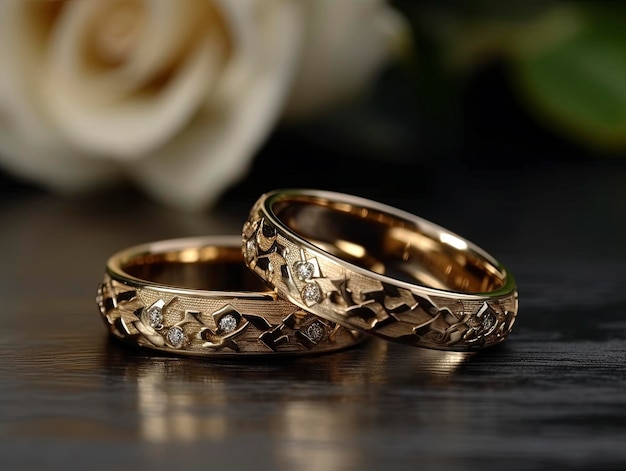This image showcases a close-up view of two intricately designed gold wedding bands adorned with diamonds. The bands, which have a bronzy gold color and both a polished and textured finish, feature detailed, raised patterns with embedded white diamonds. One ring lies flat on a brown wooden table, while the other is propped against it at an angle. In the blurred background, a cream-colored rose and some leaves can be seen, adding a romantic touch to the scene. The focus of the photo is sharply on the rings, highlighting their elaborate design and the sparkle of the diamonds.